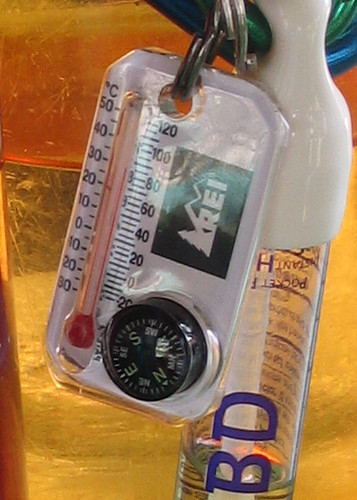The image features a packaged thermometer prominently centered. The thermometer, still within its packaging, is secured by a metallic, claw-like device resembling a keychain. The bottom end of the thermometer is bulb-shaped and red, continuing upward through a glass body with red fluid lines inside. On the left side of the thermometer, temperature markings range from 30 to -30 in increments of 10 degrees Celsius. On the right side, the thermometer displays a Fahrenheit scale from 120 to -20 in increments of 20 degrees, with "F" at the top. The thermometer's packaging includes branding with "REI" in bold white letters on a black background. The orange background likely represents a scratched table surface, suggesting a textured and possibly glass-like material at the bottom.